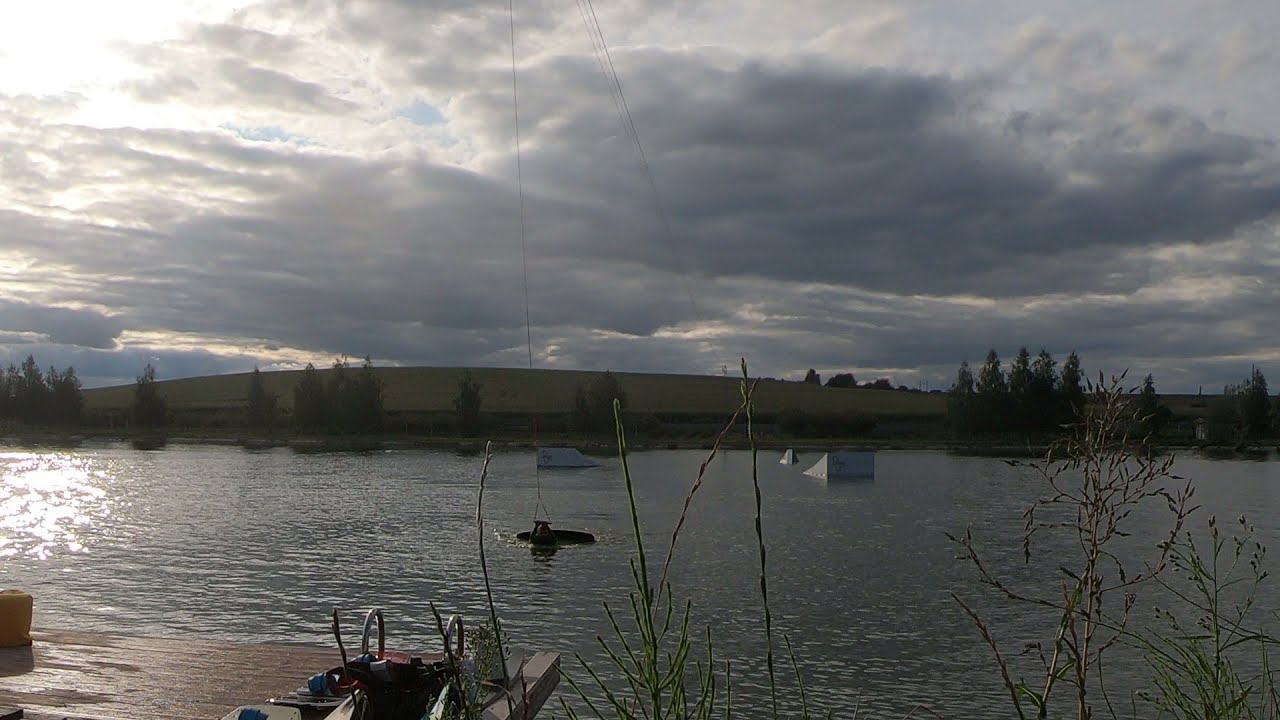The image depicts a tranquil, outdoor lake scene on a cloudy day. The sky is dominated by dark, gray clouds with only a hint of blue visible, creating a somber, low-light atmosphere. The water is calm and flat, with a grayish hue, reflecting the minimal light breaking through the clouds. Prominently in the foreground, there are plants growing near a small pier or deck that extends into the lake. Among the objects in the water, there are noticeable ramps likely for boats or water skiing, and possibly a ladder or pier structure pulled onto a sandy shore area. The lake is bordered by tall brush and larger pine trees on its far side. Additionally, a large, indistinct gray-beige building spans the background, partially obscured by the trees sprouting along the shoreline. The overall setting gives off a serene, woodsy vibe typical of an up-north lake.